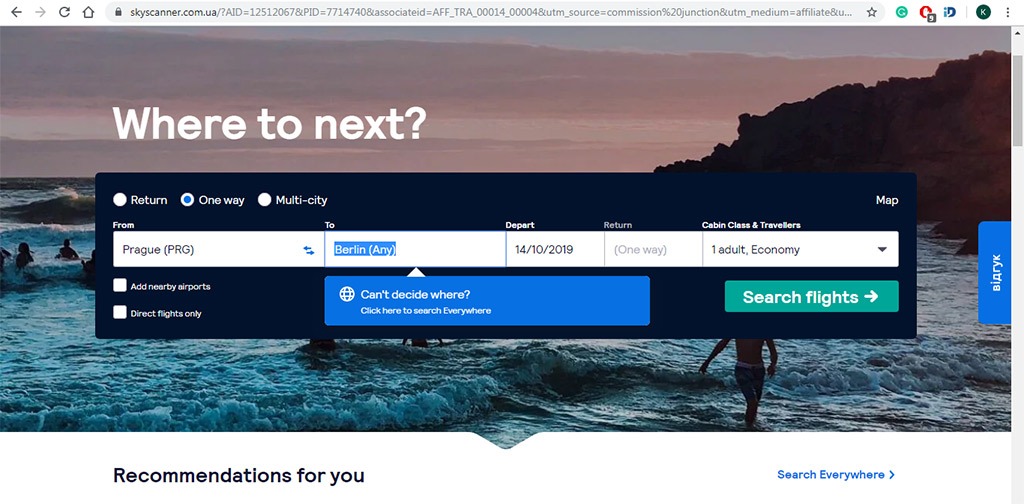This screen capture showcases the user interface of the Skyscanner website featuring various navigational and search elements. At the very top, the image displays browser navigation tools including a back arrow (clickable), a grayed-out forward arrow, a refresh icon, a home icon, a padlock symbol for security indication, and an address bar showing "skyscanner.com.ua" followed by an extensive string of letters and numbers. To the right of the address bar, there is a star icon for bookmarking, a green circle with a white arrow, a red icon next to a gray box, a blue “D” icon, a dark green and white “K” icon, and three gray dots representing additional options.

The main section of the screen features white text that reads, "Where to next?" positioned against a striking background image of people in the water. The water is a vivid blue, complementing the slightly grey sky with pink clouds. A prominent brown rock outcropping with water breaking around it and waves add to the scenic beauty. Visible participants include someone in swim trunks walking through the water.

Overlaying this image is a navy pop-up box with a mix of white and black text. The top of this box displays three white circles labeled "Return," "One way" (with a blue dot next to it indicating selection), and "Multi-city." Below these labels, users can input their trip details, including the origin ("From"), destination ("To"), departure date, and return date, as well as cabin class and number of travelers. 

In the "From" section, the departure city is listed as Prague (PRG), and the destination highlighted in blue is Berlin (BER). The departure date is marked as October 14, 2019. Notably, the trip is one-way, as indicated in parentheses. For cabin class and travelers, it specifies "One adult, Economy."

Below the trip input fields are two unchecked options: "Add nearby airports" and "Direct flights only." Additionally, there is a blue box labeled "Can't decide where? Click here to search everywhere" and a teal box with white text stating "Search flights," accompanied by an arrow icon. At the bottom of this pop-up box, it says "Recommendations for you" and another "Search everywhere" button in blue.